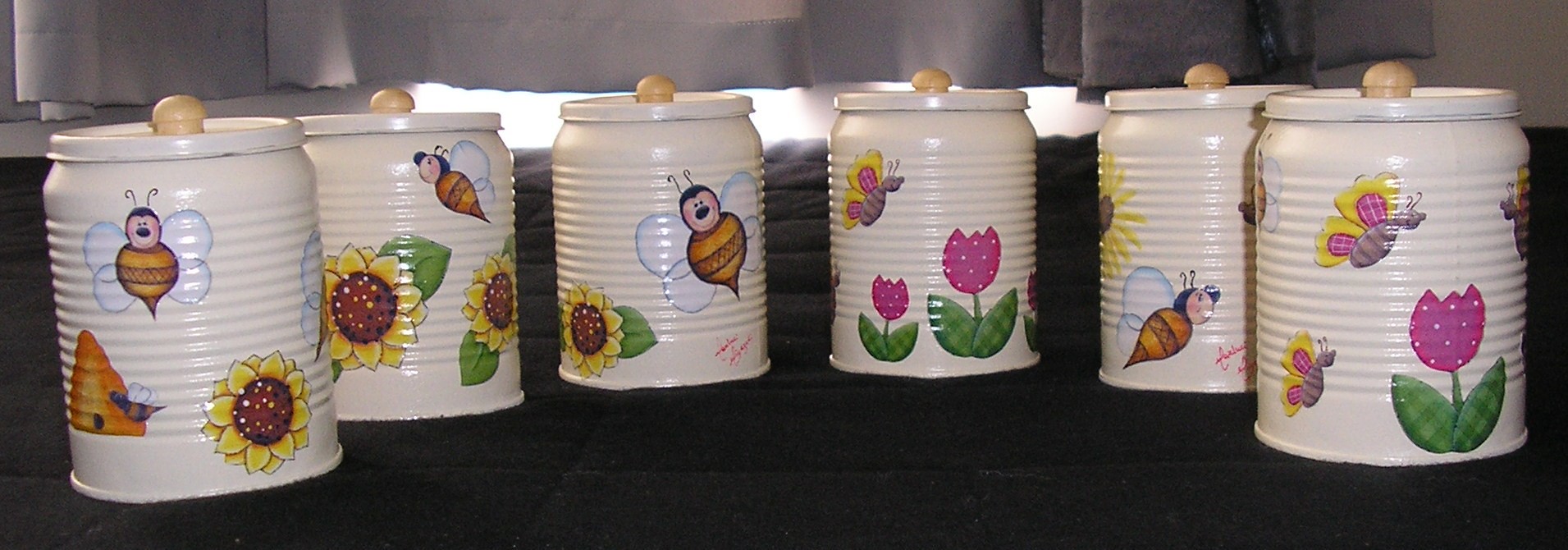The image features six identically sized white containers resembling mason jars with ridges like those on store-bought cans. Each container has a white lid topped with a brown knob. The intricately painted decorations on these jars include a variety of cheerful elements: cartoon-like bees with little faces, vibrant yellow sunflowers—some complete with green leaves—pink tulips, and butterflies on several of the jars. One jar displays a detailed beehive with a bee flying into its center. They are arranged on a black surface, possibly a countertop or table, and the background includes a gray curtain with light filtering through a window, adding a cozy ambiance to the scene. The grooved design of the containers starts about an inch from both the top and bottom, adding to their charm and texture.